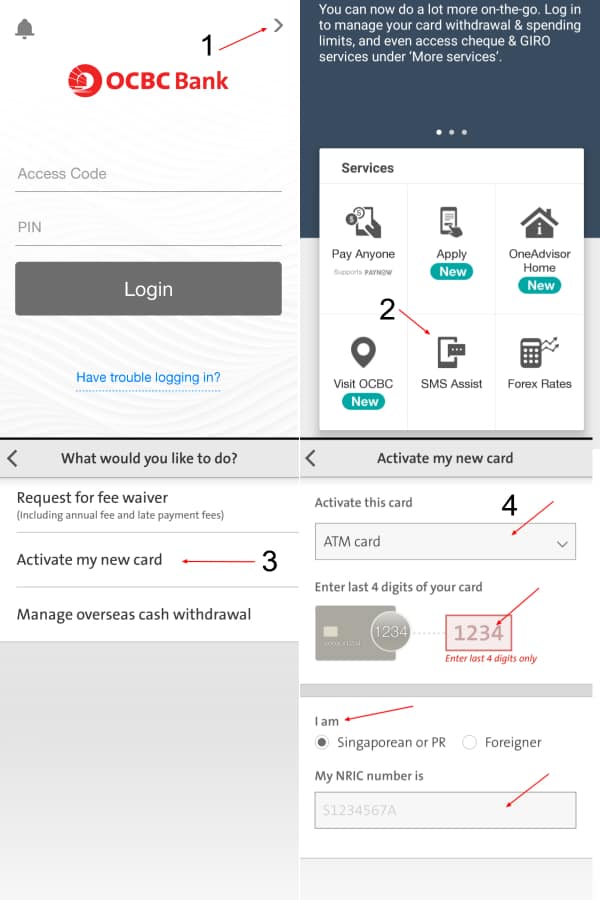The image depicts a page from OCBC Bank. Prominently, the OCBC Bank logo is positioned in the upper-left corner, featuring a bolded red font and an accompanying icon. Above the bank's name is a large red "1" with an extended arrow pointing to a clickable area, emphasizing the bank's mobile capabilities. Here, users can log in to manage their card, adjust withdrawal and spending limits, and access additional services like cheques (noted as "C.H.E.Q.U.E." indicating British English usage) and G.I.R.O. under "More Services."

Below the OCBC Bank logo, there are fields for "Access Code" and "PIN" alongside a "Log In" button. A white box within this section provides options for various services, allowing users to make payments, apply for features, and perform numerous other tasks.

Additionally, a grey section at the bottom, with black text, asks users "What would you like to do?" and offers instructions for activities such as activating a new card, guiding users through the necessary steps to log in and get started with their banking needs.